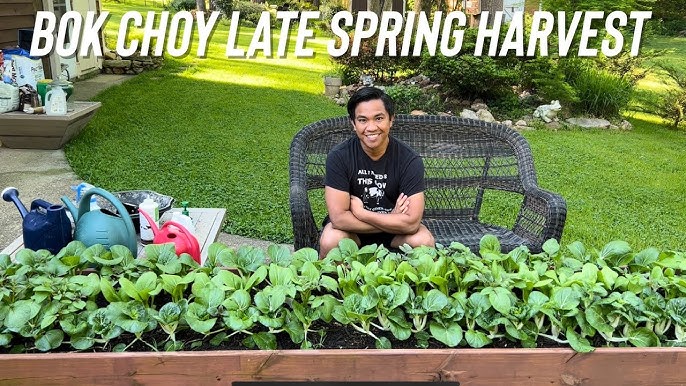A man is sitting on a large dark brown rattan bench, smiling proudly at the camera. He is wearing a black t-shirt and black shorts. In front of him, there is a healthy bed of green bok choy plants growing in a polished wooden framed nursery bed, clearly well-cared for. Beside him, to the left, are three watering cans in red, blue, and dark blue. In the background, a lush green lawn stretches out, adorned with bushes and a circular decoration made of flowers and stones. The scene is topped with white lettering that reads "Bok Choy Late Spring Harvest," indicating that this image is likely a YouTube thumbnail for a gardening video about harvesting bok choy. The setting also includes a small area where gardening supplies like chemicals and soil are kept.